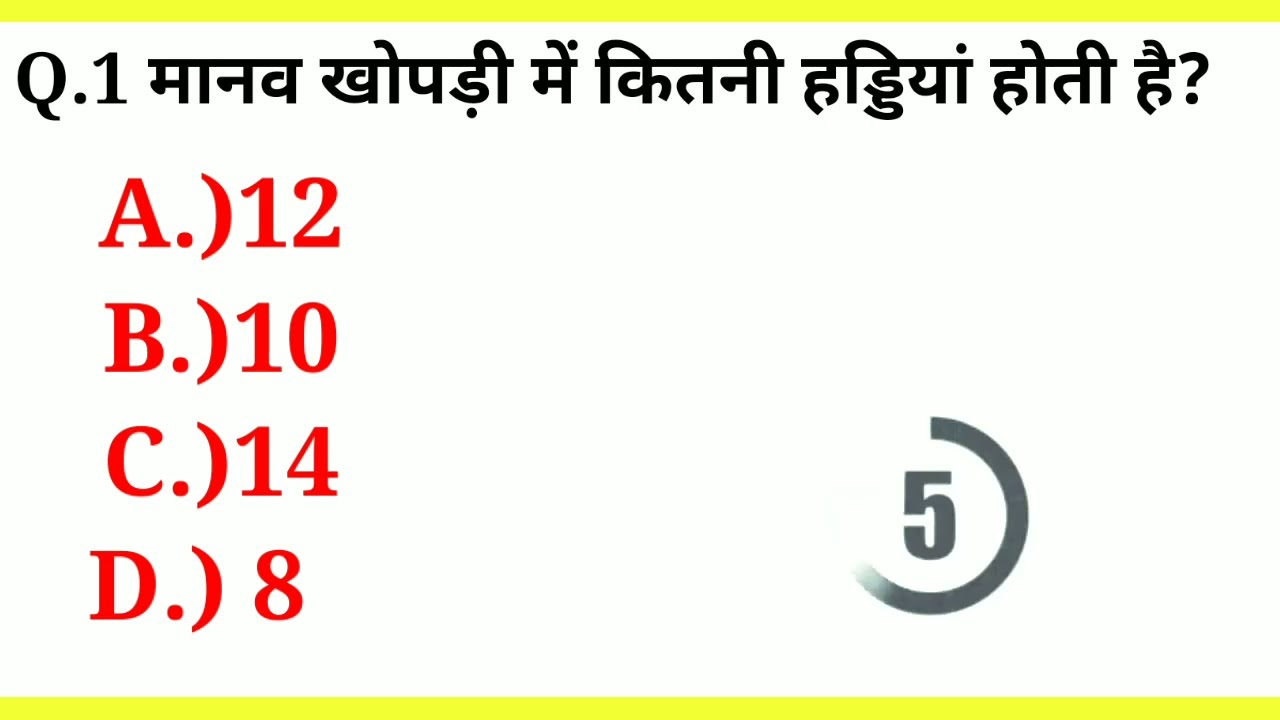The image features a predominantly white background framed by thin yellow bars at the top and bottom. In the upper left-hand corner, just below the top yellow bar, there is black text that begins with "Q1," followed by characters that appear to be Asian and ending in a question mark. Below this text, the answers are listed vertically in red, each on a separate line: "A12," "B10," "C14," and "D8." On the right side of the image, near the bottom, there's a gray number "5" encircled by an incomplete, thick gray semicircle, indicating a countdown timer. The scene appears to depict an electronic quiz program interface.